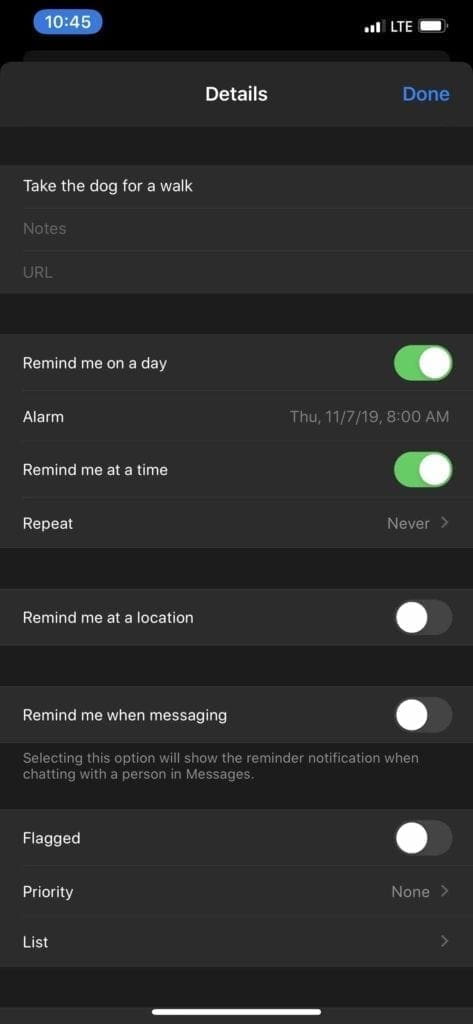This is a detailed screenshot from a cell phone, serving as a visual documentation of a reminder setup. At the very top, the status bar displays the current time, "10:45," highlighted in blue, accompanied by icons indicating a nearly full battery and strong Wi-Fi signal. 

Below the status bar, the screen reveals a detailed view of a reminder created in the reminders app. The header reads "Details," with a "Done" button adjacent to it. The main content starts with the reminder text, "Take the dog for a walk." 

Following that, there are various customizable options for setting the reminder. An option for adding "Notes" and "URL" is present. The "Remind me on a day" option is highlighted in green, specifying that the alarm is set for Thursday, November 7, 2019, at 8:00 a.m. The "Remind me at a time" option is also selected. 

Other options include "Repeat," set to "Never," "Remind me at a location," and "Remind me when messaging," both of which are not selected. There is a note explaining that selecting the messaging reminder option will display a notification when chatting with a person in messages. 

Additionally, there is an option to mark the reminder as "Flagged," which is not selected, and set a "Priority," currently indicated as "None." Finally, a "List" option featuring a right-facing arrow is displayed, possibly leading to further customization or sorting options.